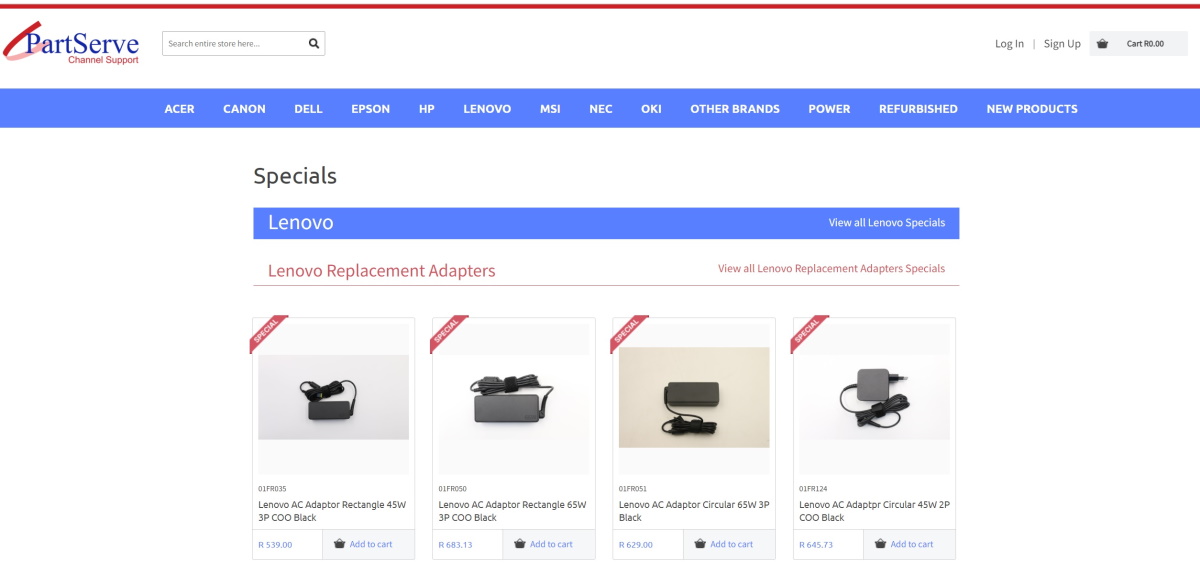The shopping website features a clean and simple design, prominently showcasing products and brands. Starting from the top left corner, there's a blue logo with a distinctive red slash, displaying the name "PartServe" (with a capital 'P' and 'S,' all one word). Beneath the logo, in small red letters, is the tagline "channel support."

A blue banner stretches across the top of the page, listing various computer and printer brands in white text, such as Acer, Canon, Dell, Epson, Lenovo, MSI, and NEC. 

At the center of the page is a "specials" section. This area has a blue banner with the brand name "Lenovo" in white letters. Below this, in red text on a white background, the category "Lenovo replacement adapters" is displayed. Four different Lenovo replacement adapters are showcased as thumbnails, each featuring a red banner with white text reading "special" across the upper left diagonal corner of the thumbnail. All four adapters are visually similar, indicating they're part of a special promotion.

Overall, the page is well-organized with a focus on brand visibility and highlighted specials.